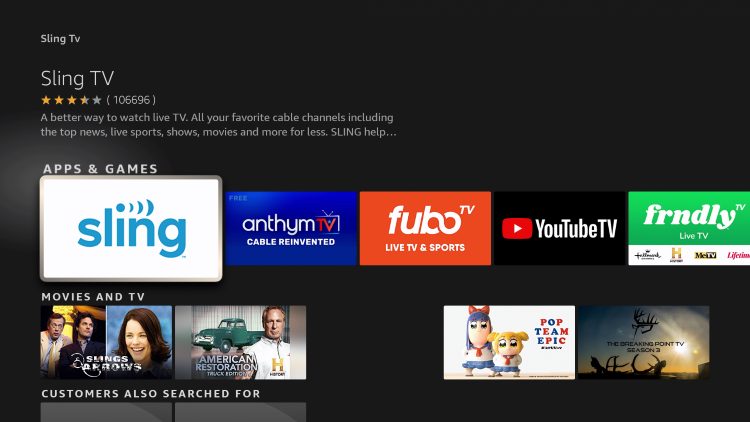The image is a horizontally oriented rectangle with a dark gray to black background. In the top left corner, the words "Sling TV" are written in small white text. Just below, the "Sling TV" logo appears again, slightly larger. This is followed by a rating of four and a half stars out of five, based on 105,695 reviews. Below the ratings, there's a tagline that reads, "A better way to watch live TV—all your favorite cable channels, including top news, live sports, shows, movies, and more for less," accompanied by the URL slinghelp.com.

In the middle-left section of the image, under the category "Apps and Games," the Sling app is highlighted. To the right of it are logos for other streaming services: Anthem, Cable Reinvented, Fubo, Live TV and Sports, YouTube TV, and FRNDLY Live TV.

On the lower row, under "Movies and TV Shows," partially visible icons include titles such as "American Restoration" and "Pop Team Epic," amongst others that are not clearly readable.